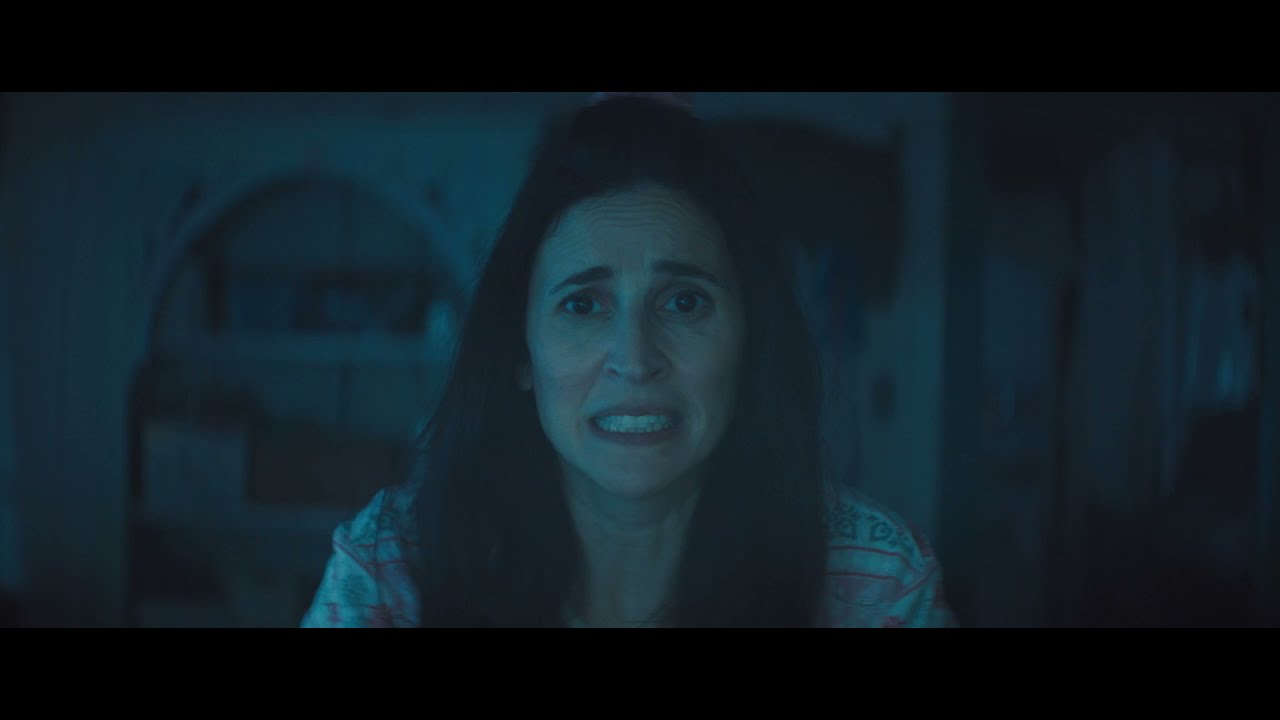The image depicts a woman indoors, possibly inside a house, enveloped in a greenish-teal hue. Her dark, straight hair falls past her shoulders, and she has prominent dark eyes and eyebrows, which are raised as if in distress. Her expression exudes fear; her mouth is slightly open, clenching her teeth, revealing her white teeth, and her eyes are wide with concern. She wears a light-colored shirt adorned with bright patterns and stripes. The setting appears dim and shadowy, as if it’s nighttime. Behind her, to the left of the image, is a blurry built-in shelf with indistinguishable objects. Additionally, there's a hint of a light switch and maybe some doors or windows further illustrating the indoor environment. The woman is centered in the image and looks directly at the camera, amplifying her terrified expression as if reacting to something alarming out of view.